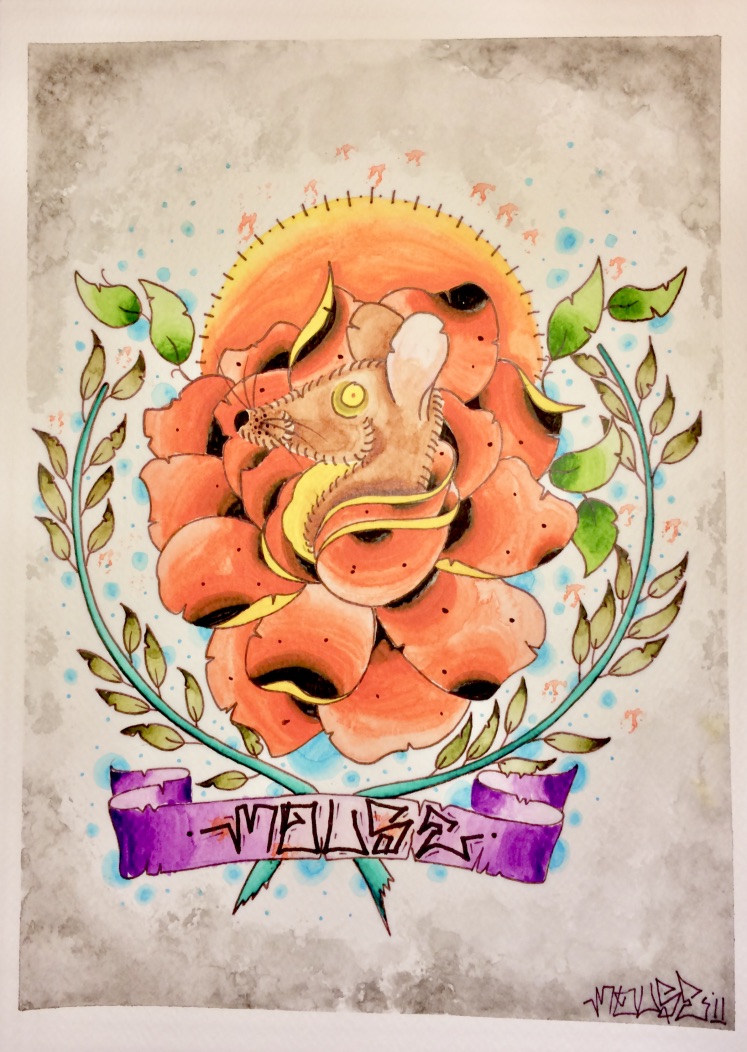This intricate drawing features a mouse centered on a pinkish beige background. The mouse is predominantly brown with a yellow belly and a distinctive yellow eye, and it faces to the left. It has well-defined whiskers that add to its detailed features. Surrounding the mouse are vibrant orange petals, resembling a flower in full bloom. Above the mouse and flowers, an orange globe, possibly representing the sun, rises, adding warmth and depth to the scene. Encircling the orange petals is a lush, twisting green and blue vine, adding a natural frame to the composition. Beneath the mouse, a purple ribbon, adorned with indistinct writing, adds a final touch of mystery and elegance to the artwork.